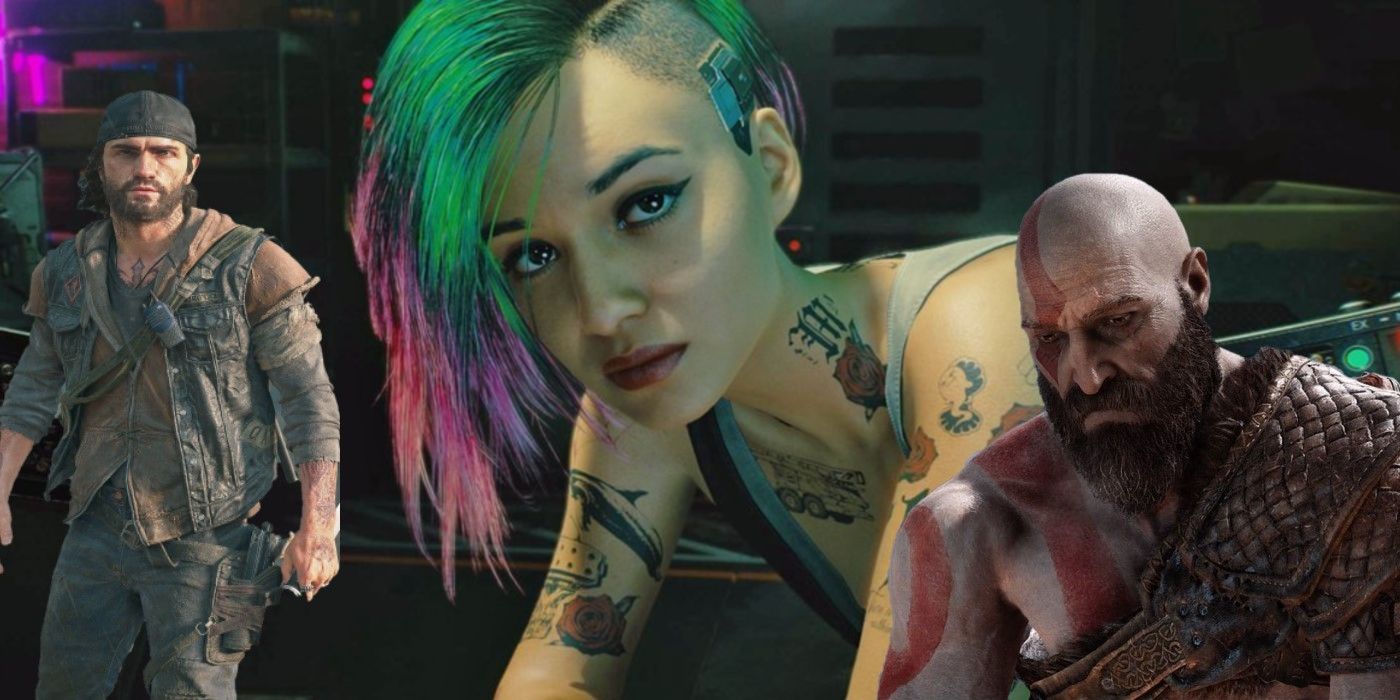The image depicts a trio of distinct 3D characters, evoking a modern video game aesthetic. Central to the composition is a striking cyberpunk woman in her early 20s with edgy, green hair that fades into pink at the ends, shaved on one side to reveal mechanical components. She sports a tank top, with bold black tattoos, including roses, adorning her arms and extending to her long neck. Her makeup is equally striking, with noticeable lipstick and eyeliner.

Flanking her on the right is a character unmistakably reminiscent of Kratos from the God of War series. His skin is an ashen white, punctuated by a rugged brown beard with streaks of gray. He wears minimal armor, primarily covering his left shoulder, and is marked with distinctive red tattoos that trail down his face, chest, and shoulders.

On the far left stands a grizzled, tough-looking man, emitting a fighter's aura. He dons a black cap or do-rag, a long sleeve shirt, and a rugged, multi-pocket cargo vest paired with cargo pants. A gun holster completes his combat-ready ensemble.